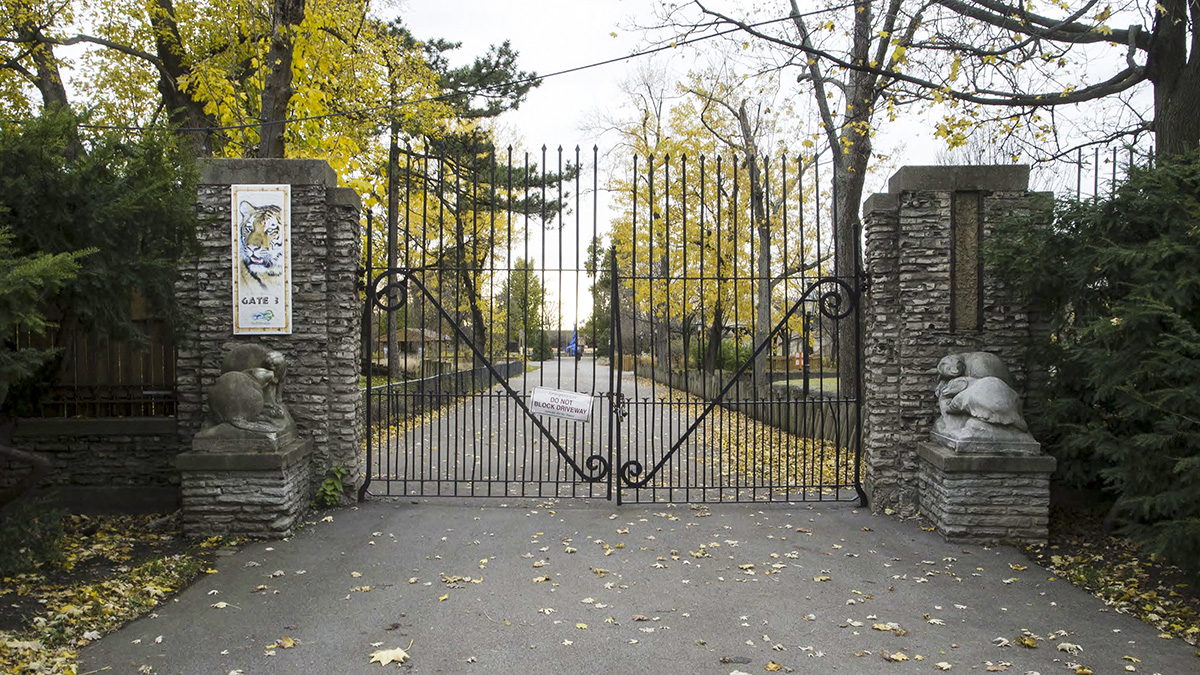This color photograph captures a closed, imposing iron gate which appears to serve as an entrance to a significant site, possibly a zoo or a large estate. The gate is black, approximately 12 feet high, and features pointed edges along the top. It consists of two halves that swing open in the middle. The gate's frame is flanked by two approximately 10-foot high stone pillars, crafted from stacked bricks. Each pillar is topped with stone or cement sculptures resembling animals, though their exact species is unclear. On the left pillar, there's a sign that seems to read "Gate 1", adorned with an illustration of a lion's head above it. The road leading to the gate is an asphalt road, scattered with yellow and red fallen leaves and lined with trees, some of which are already bare. The road is just wide enough for a single car to pass. Beyond the gate, the path continues, bordered by more trees and small walls, and eventually leads to visible buildings and structures in the distance.